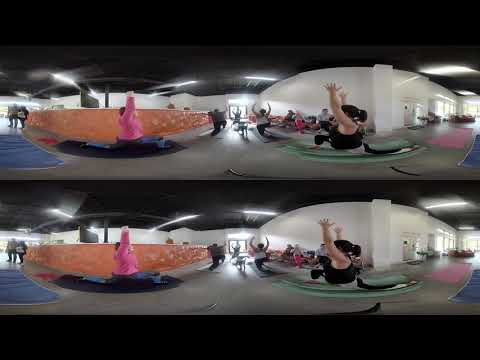In an indoor exercise studio, the picture features a duplicated, mirrored image divided horizontally into two identical parts. The scene, captured with a curved perspective, shows individuals participating in a yoga session. On the left side of both the top and bottom halves, a woman in a pink long-sleeve shirt and dark pants stands on a black mat with her arms raised. Behind her, the peach-colored wall is visible, along with several other participants scattered around the studio. On the right side, a woman in a black sleeveless top and black-and-white yoga pants also has her arms raised, standing on a green mat. There are additional yoga mats of various colors, including red and blue, scattered across the floor, indicating the presence of more participants engaging in the session. The black ceiling and the well-lit space contribute to the ambiance of this health center setting.